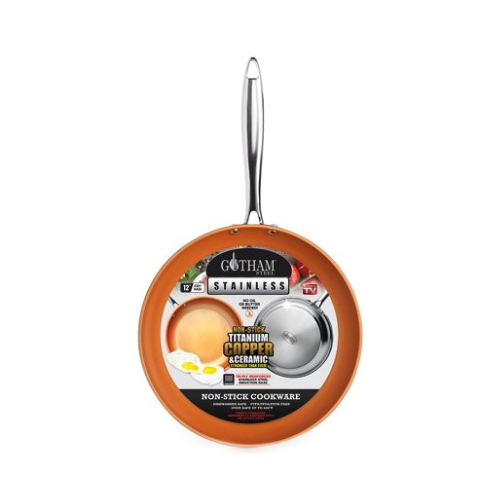This image captures a detailed top-down view of a 12-inch stainless steel frying pan, also known as a skillet, with a silver handle pointing upwards. The handle, featuring a hole for easy grasping, seamlessly transitions into the pan's elegant copper-colored interior, while the bottom is a contrasting stainless steel. The base of the pan still retains its information sticker, displaying the brand name "Gotham" in insular writing on a black bar with a silver strip below it. The sticker highlights this item as a titanium, copper, and ceramic non-stick cookware. Additionally, the sticker features two photographs: on the right, a chrome frying pan, and on the left, a silver frying pan showing its bottom side. There is also an image of two fried eggs frying in a copper skillet. The pan appears to be in a hanging position, possibly displayed in a store, and stands out as a versatile, aesthetically pleasing piece of cookware ideal for various kitchen tasks.